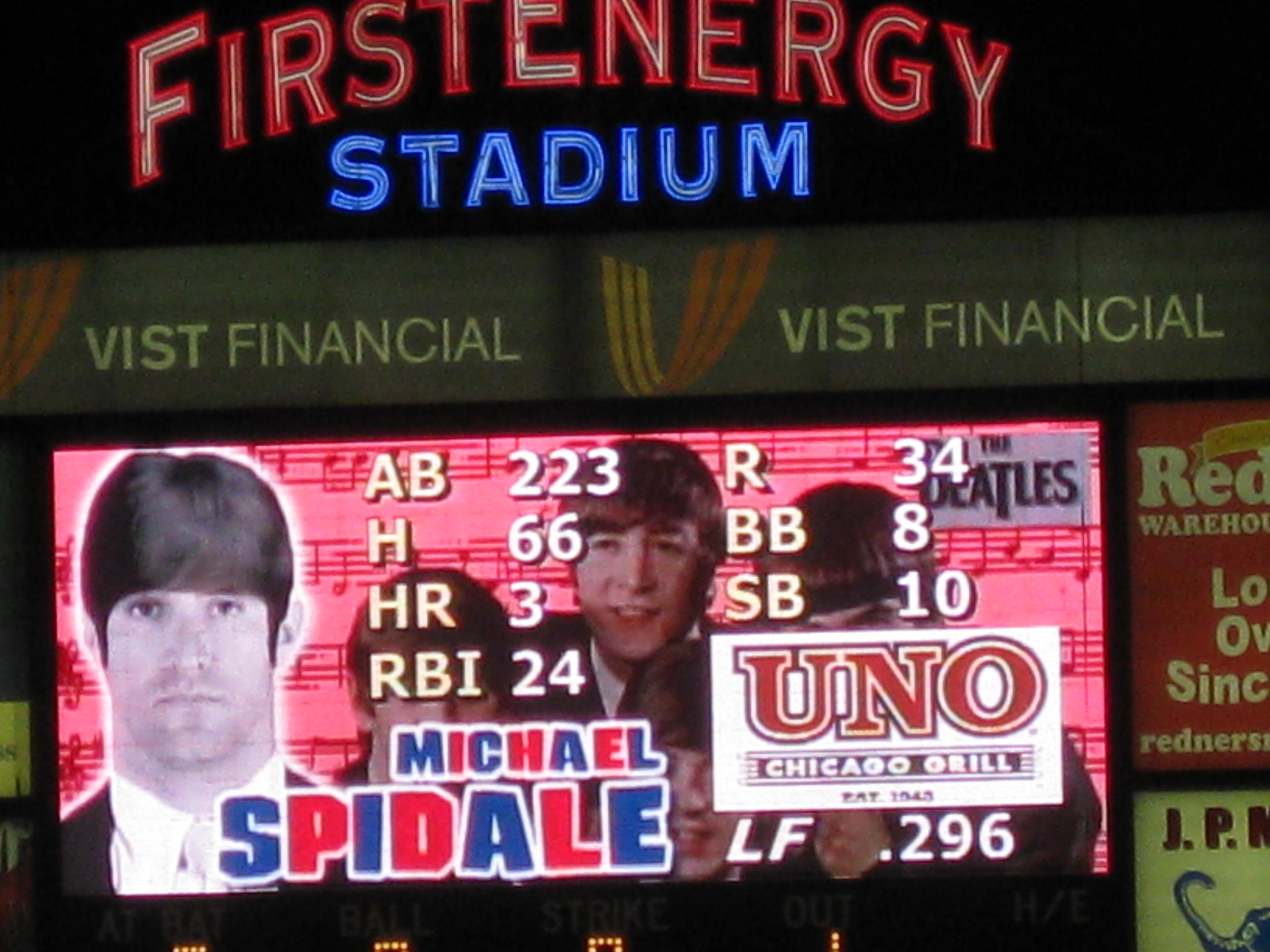The image is a horizontally rectangular poster designed to resemble a scoreboard from a baseball stadium, captured at night. At the top, the neon-lit words "FIRST ENERGY" in red and "STADIUM" in blue are partially cut off by the image's upper edge. Below this, there is an advertisement in green with the repeated text "VIST FINANCIAL.” 

The primary feature of the scoreboard is a visually striking promotional graphic displaying baseball player Michael Spadale, whose name is styled in alternating red and blue bubble letters. The graphic shows two images of him, one with a Beatles-themed twist: Michael is either photoshopped or dressed in a mop-top wig and suit, reminiscent of the iconic band members, against a background of pink with black musical notes.

Accompanying his images are career statistics, including his position as a left fielder and a .296 batting average. The right portion of the scoreboard includes an advertisement for Uno Chicago Grill on a white background, while another indistinct red ad occupies the bottom right-hand corner. Additionally, the upper right-hand corner features Beatles imagery, further contributing to the theme's integration into the design.